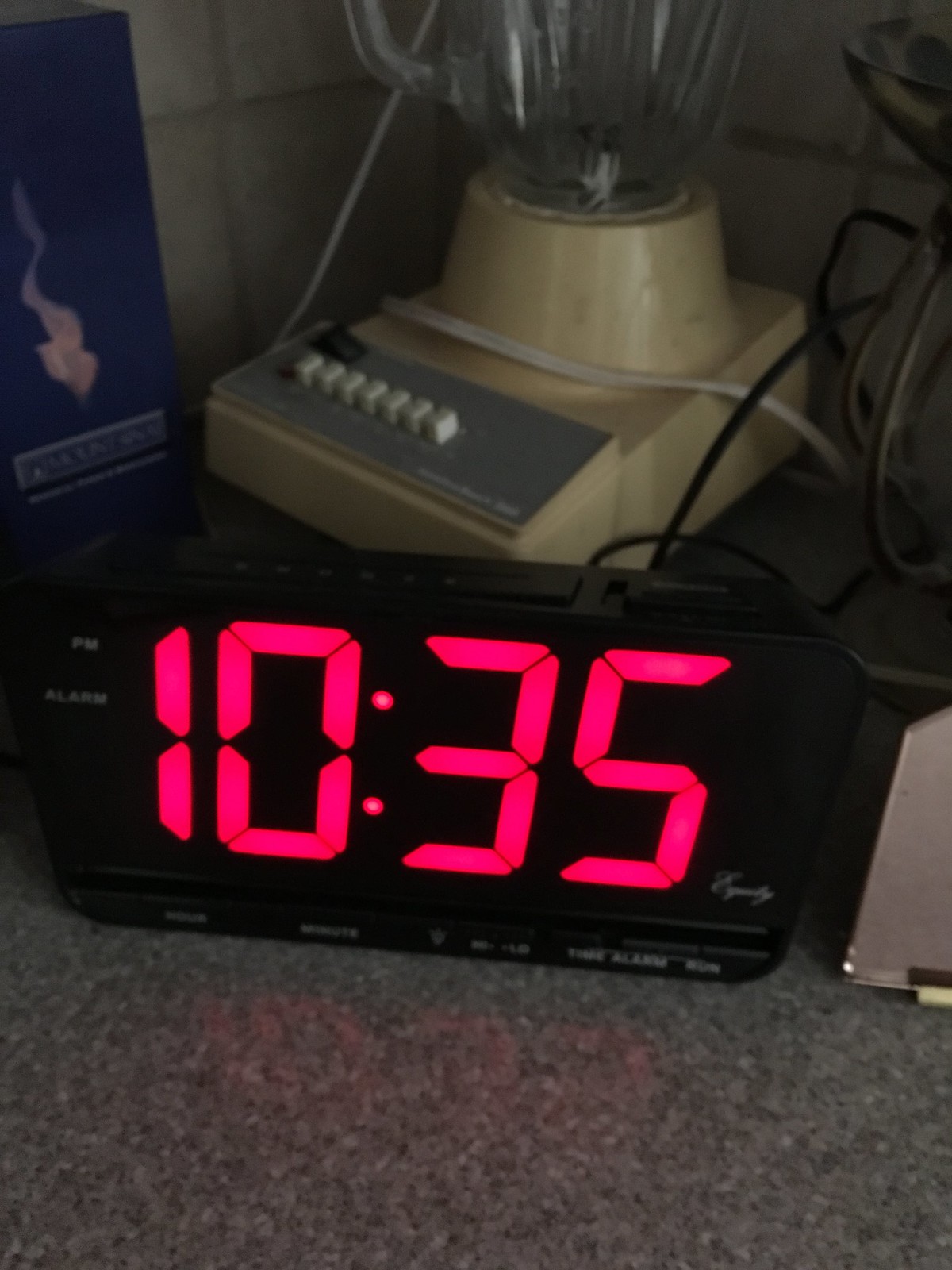The image features a sleek, black pyramidal digital clock prominently displaying the time 10:35 in large, bright red numbers. The clock is positioned horizontally on a polished granite countertop. In the background, an avocado green blender with a multitude of white buttons and a glass container is situated on the counter. The blender's white electric cord is visible. Behind the blender is a rectangular-shaped backsplash composed of white tiles arranged in a brick pattern, adding a clean and modern touch to the kitchen scene.